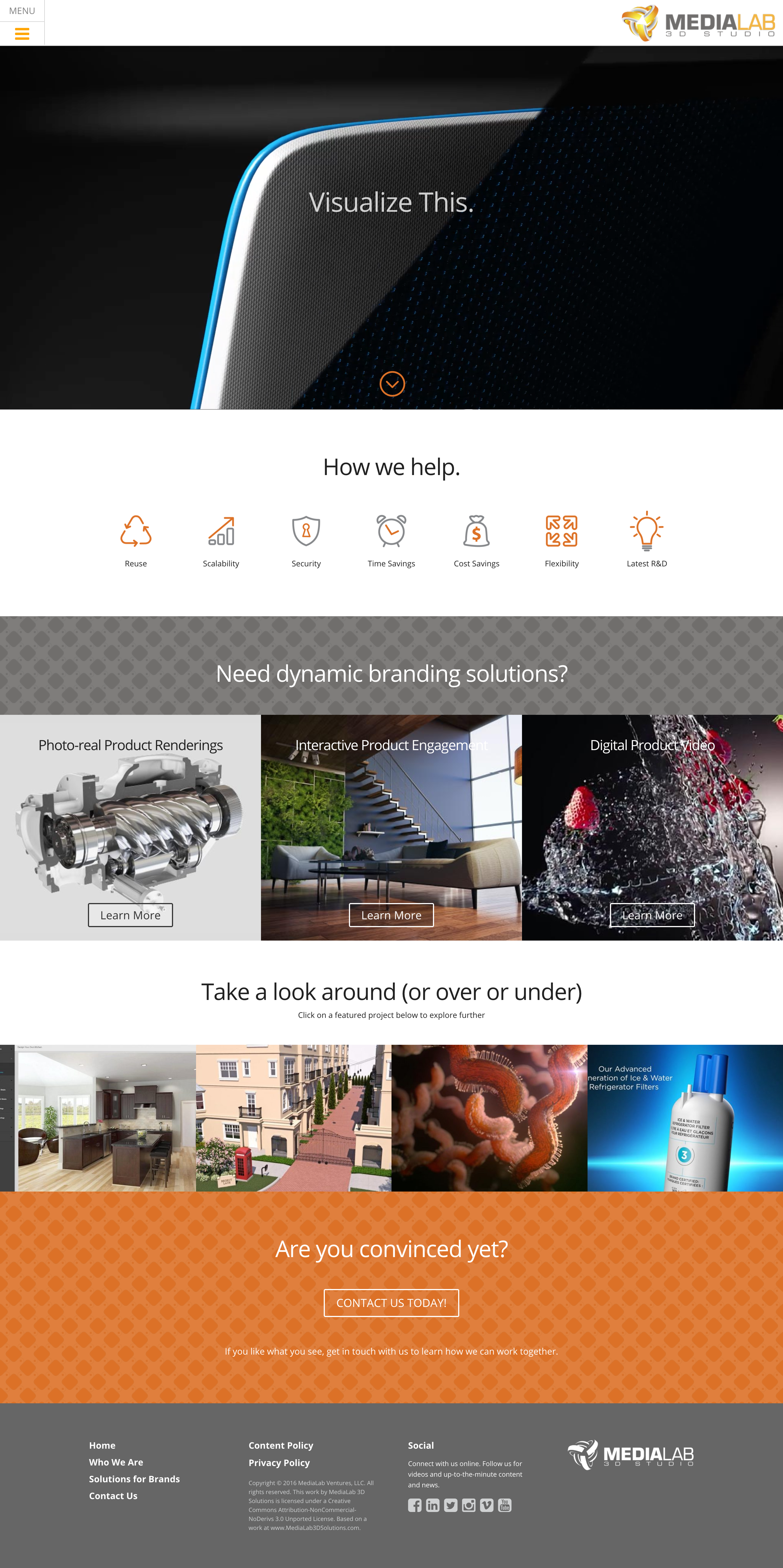This photograph captures a detailed snapshot of the Media Lab website. The header prominently features the text "Media Lab," with "Media" in black font and "Lab" in yellow. To the left of this text, there is a distinctive yellow triangle logo. The layout of the website is organized into three primary rectangular sections. 

The top section features the headline "Visualize This," providing an inviting introduction. The middle section is focused on their services, asking, "Need Dynamic Branding Solutions?" and highlighting their expertise in creating impactful branding. The bottom section includes a call to exploration with phrases like "Take a look around, over, under," and "Are you convinced yet?" which encourages further interaction with their content.

The imagery on the website includes clip art and stock photos, such as an outline of a smartphone and generic modern office scenes, featuring wood flooring and contemporary furniture. The website's color scheme predominantly uses a clean combination of white and black, with accent colors including blue, orange, gray, and silver. 

At the bottom of the page, the Media Lab logo appears alongside links to their social media profiles, reinforcing their presence and connectivity. Overall, the website effectively markets Media Lab as a professional branding and web marketing company.